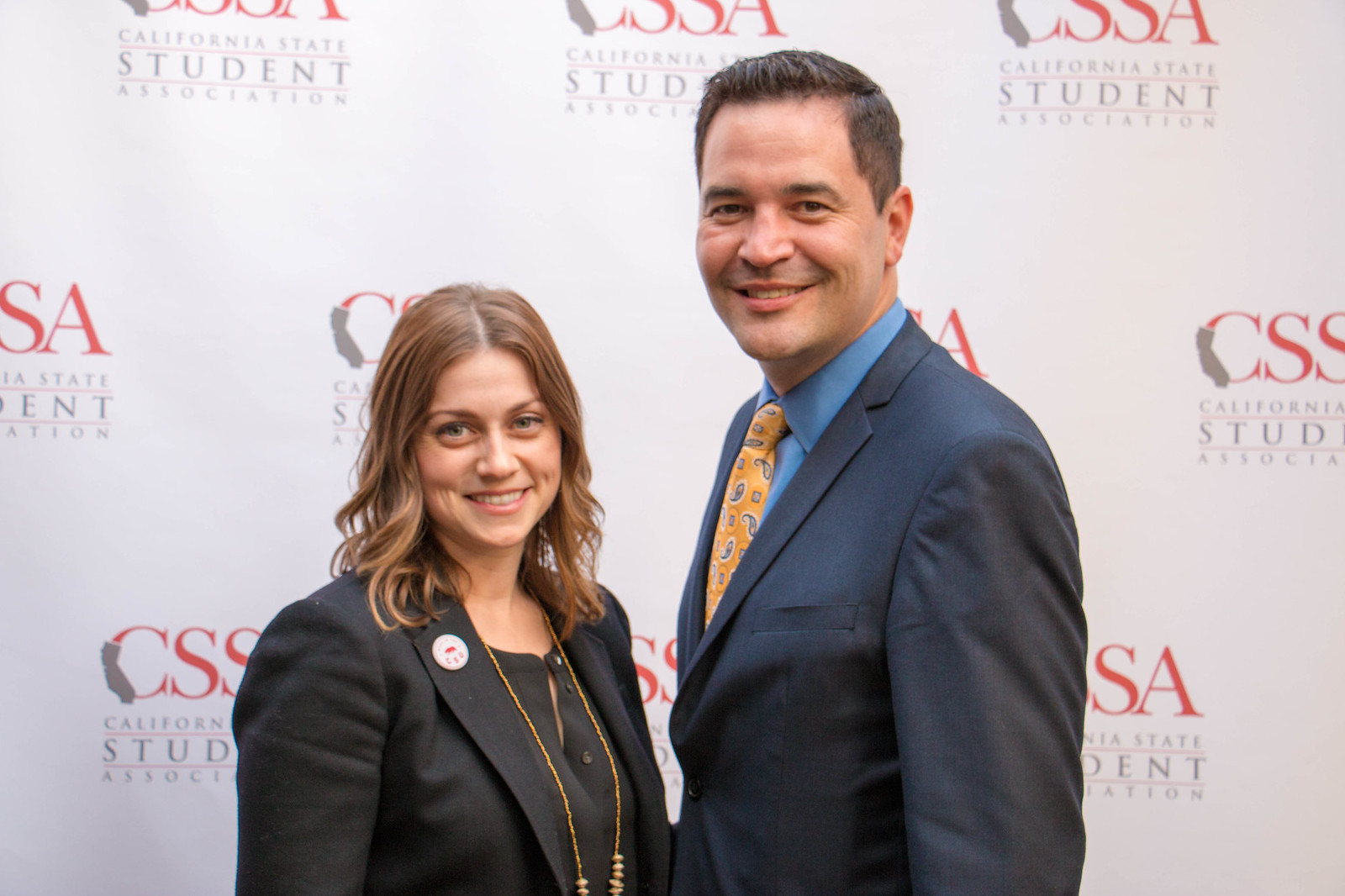In this wide rectangular image, two individuals are smiling in front of a backdrop adorned with a repeating logo. The logo features large red letters “CSSA” with a gray outline of California over the "C", and below it, in gray letters separated by red lines, it reads “California State Student Association.” The background is predominantly white, enhancing the prominence of the logo.

On the left is a young woman with somewhat curly red hair, dressed in a black button-up shirt, a black blazer, and a long gold necklace. She also has a pin on the collar of her blazer. To her right is a taller man with light skin and short cropped brown hair. He is dressed in a brightly blue button-up shirt paired with a navy blue blazer and a distinctive tie with yellow and purple patterns. Both are smiling warmly and looking directly at the camera.